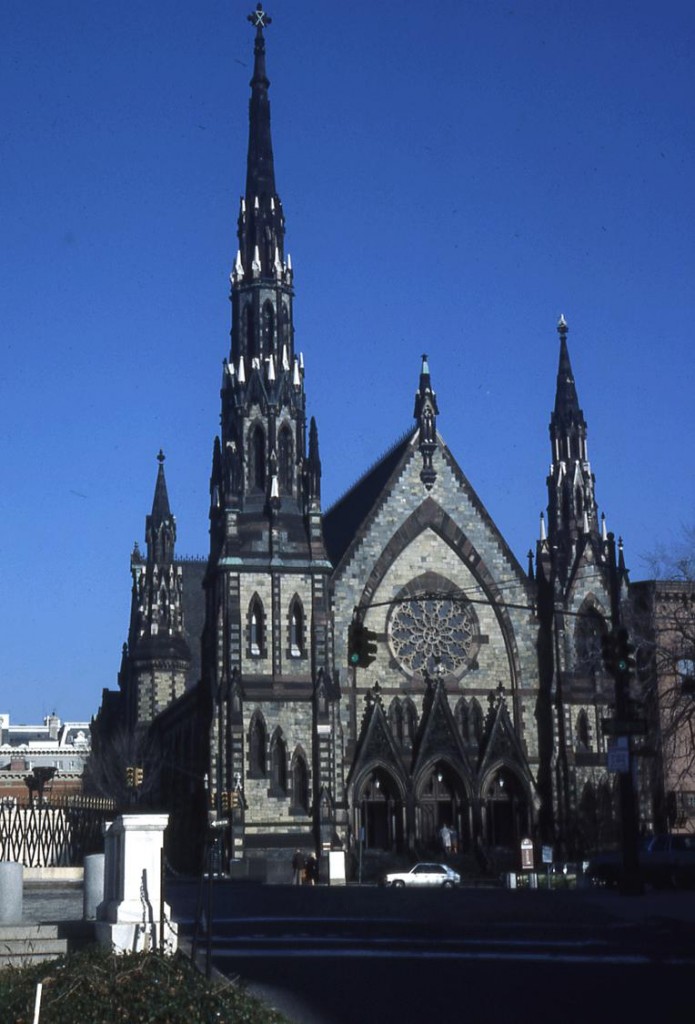This detailed image captures a grand cathedral taken from across the street under a clear, blue sky. Dominating the foreground, the cathedral features a striking contrast between its darker stone spires and lighter gray stone facade. The most prominent element is the towering spire to the left of the main entrance, which is adorned with intricate ornamentation and smaller, white-painted spires embellishing its three distinct layers. In the backdrop, two shorter spires echo the same decorative style, adding to the imposing verticality of the structure.

The facade of the cathedral is richly detailed with a large, round stained glass window above the entrance, showcasing a floral repeating pattern that evokes natural motifs. Beneath this window, tall, arched doors—each approximately 12 feet high and crowned by steepled arches—invite entry into the cathedral. The entryway is framed by a black gated fence and concrete steps that lead up from the street level.

Numerous smaller, pointed crenellations rise from various parts of the building, contributing to its majestic silhouette. Below the grandeur of the cathedral, a small silver Hyundai and another white car are parked, providing a modern contrast against the historic and ornate architecture.